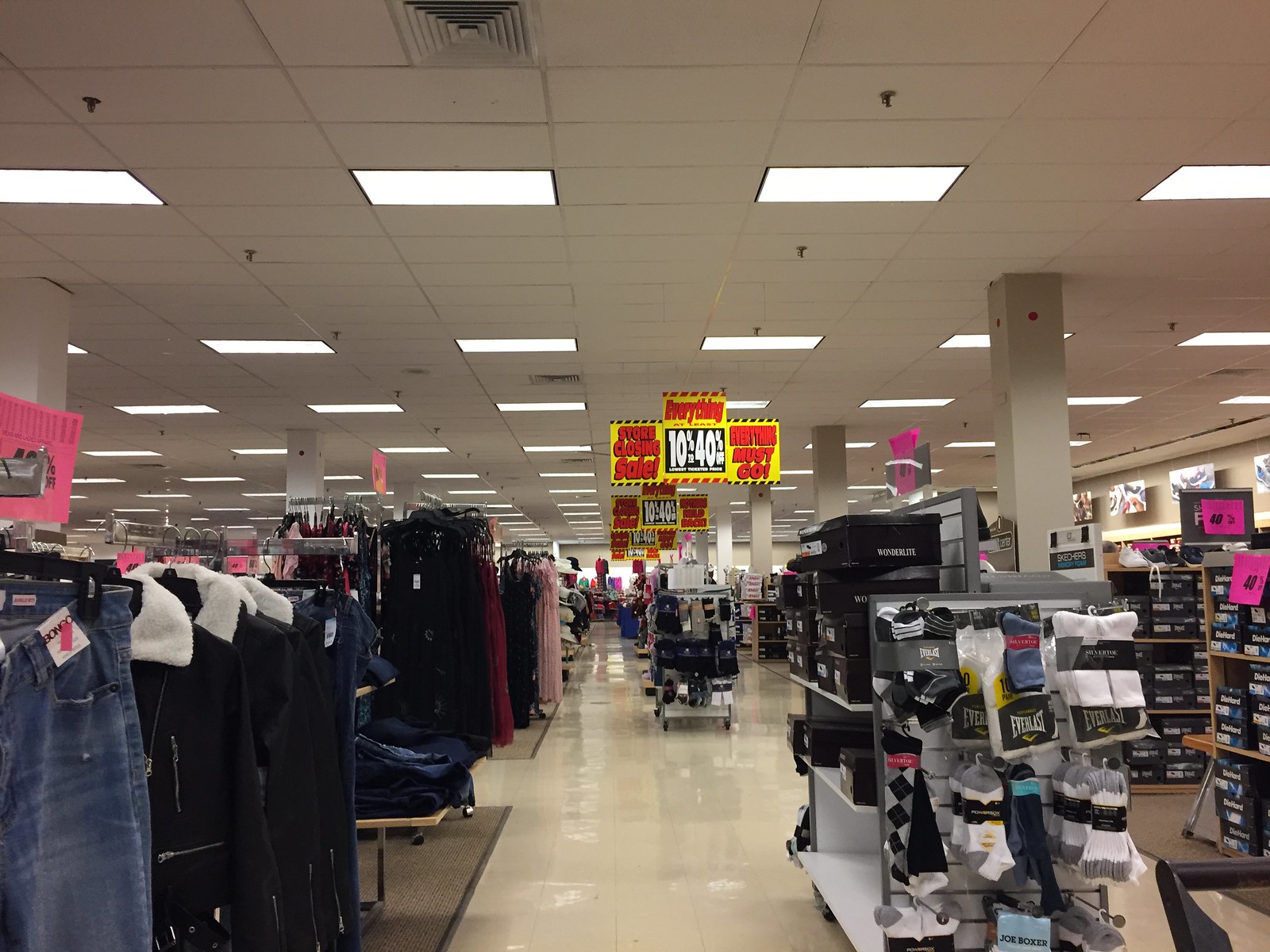The image depicts the interior of a department store that is in the process of closing down. The store has a meticulously organized layout, despite an overall sense of disarray. Prominent signs indicating a "Store Closing Sale" with discounts ranging from 10% to 40% off are strategically positioned throughout in striking pink, yellow, and red colors. These signs, including large billboards hanging from the ceiling, are intended to attract attention to the final sale event with messages like "Everything Must Go."

The store's ceiling features white tiles with rectangular lights placed in a regular pattern, providing a bright ambiance. There are also white pillars supporting the ceiling. The store's floor is beige, adding to the neutral color scheme.

In the image's foreground, Everlast socks and various shoes are displayed, with shelves of boxed shoes clearly visible. To the left are racks of denim jeans and jackets, including some with fur collars. Farther back, a section dedicated to longer gowns, such as prom or formal dresses, is visible. The right-hand side of the store mainly features shoes, with displayed signage on top of different clothing items, indicating their discounted prices after the markdowns.